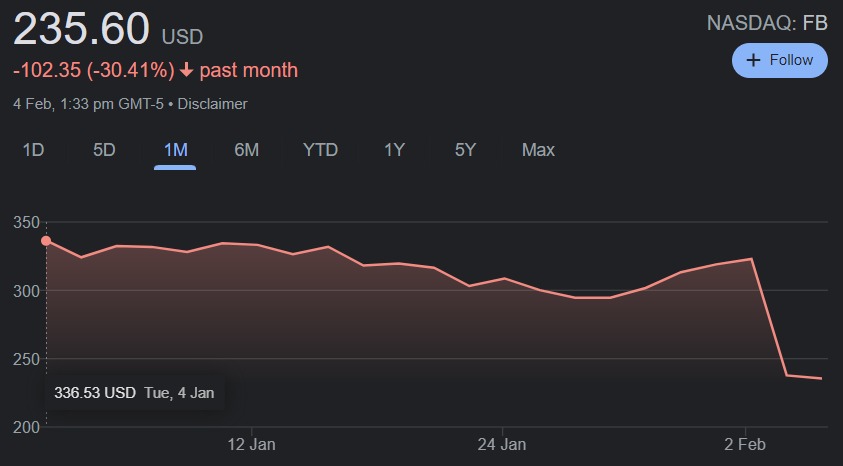The image displays a detailed stock market graph set against a black background. In the top left corner, bold white text shows the value "$235.60 USD." Directly beneath this, red text indicates a decline with the figures "-$102.35," followed by the percentage decrease "( -30.41%)" and a downward-pointing arrow highlighting the past month's performance. Below this information, in smaller gray text, the date and time are given as "February 4th, 1:33 PM GMT-5" with a "disclaimer" note nearby.

Further down, a navigation bar features various timeframes: "1D, 5D, 1M, 6M, YTD, 1Y, 5Y, and Max," with "1M" highlighted in light blue, indicating the selected period. The main graph extends below this bar, charting stock performance; the vertical axis on the left is labeled with numbers ranging from 350 to 200, while the horizontal axis at the bottom marks dates from "January 12th" to "February 2nd."